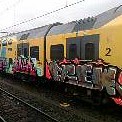The image depicts a small, detailed scene of a yellow train situated on a set of railroad tracks during the daytime. The train features multiple cars, with one prominently labeled with the number 2. The cars boast a distinctive graffitied exterior, adorned with an array of hues including predominant grays, blacks, pinks, and some splashes of red and white. The graffiti spans across each door, although the exact words are undecipherable. The train cars have gray doors, black windows, and a mix of black and gray on the roofs. The visible track, located to the left of the train, appears dark and heavily shadowed, possibly with gravel alongside it. The top section of the train car is white, further highlighting the stark contrast of the colorful graffiti against its yellow body.